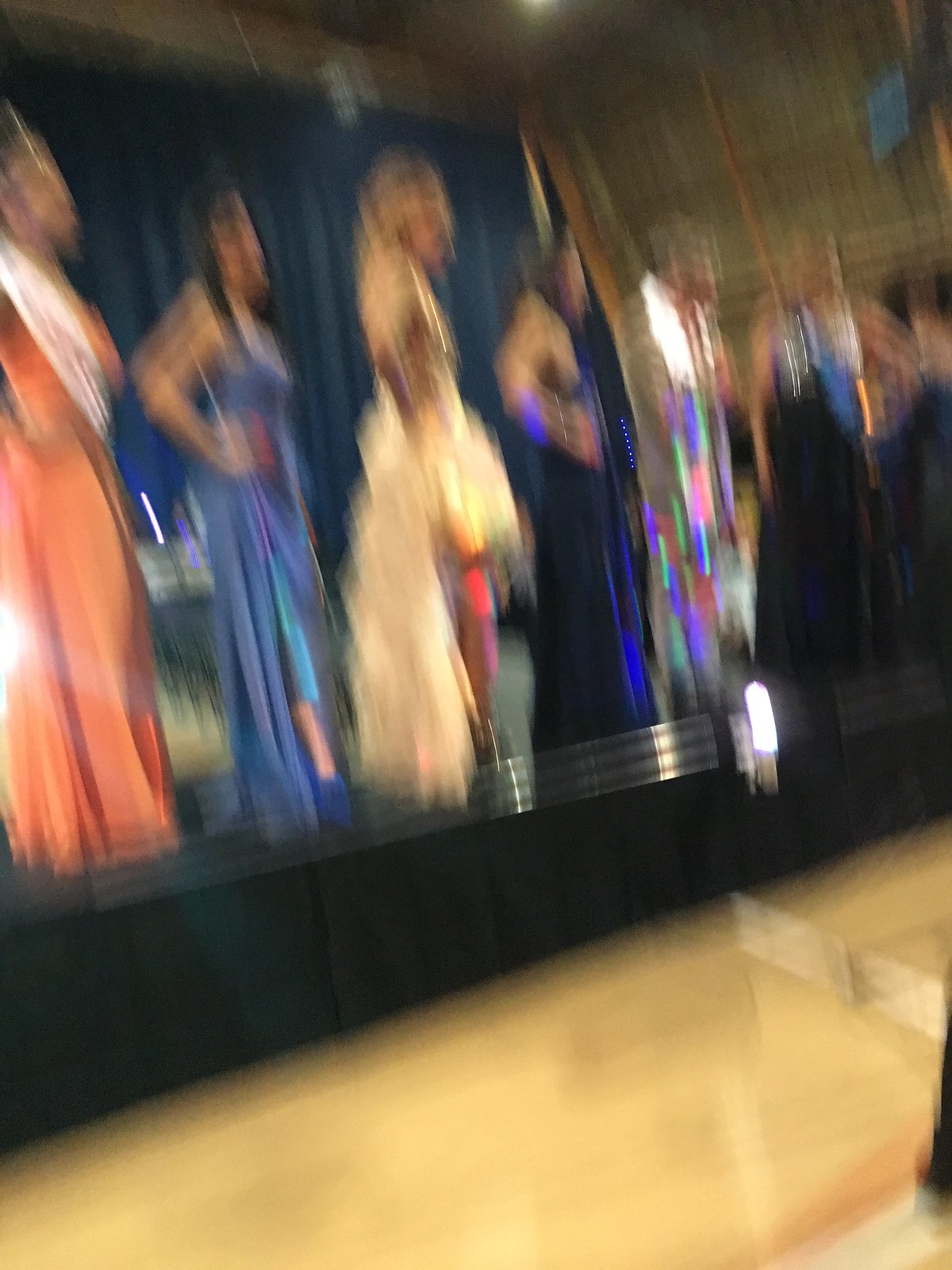The image is a blurry, first-person perspective of what appears to be a beauty pageant taking place in an auditorium or gymnasium. The entire scene is obscured as if the photo was taken in motion. In the background, there is a thin, black stage with a short silver railing. A group of women in various colored dresses are posed on the stage, all facing towards the right at about a 45-degree angle. From left to right, the women are wearing an orange or beige dress with a white sash, a thin blue dress, a puffy beige dress, a thin black dress, a shiny sequin dress, and another black dress. Behind the women, there is a long blue curtain. The floor of the auditorium is made of glossy wood, typical of a gymnasium setting.